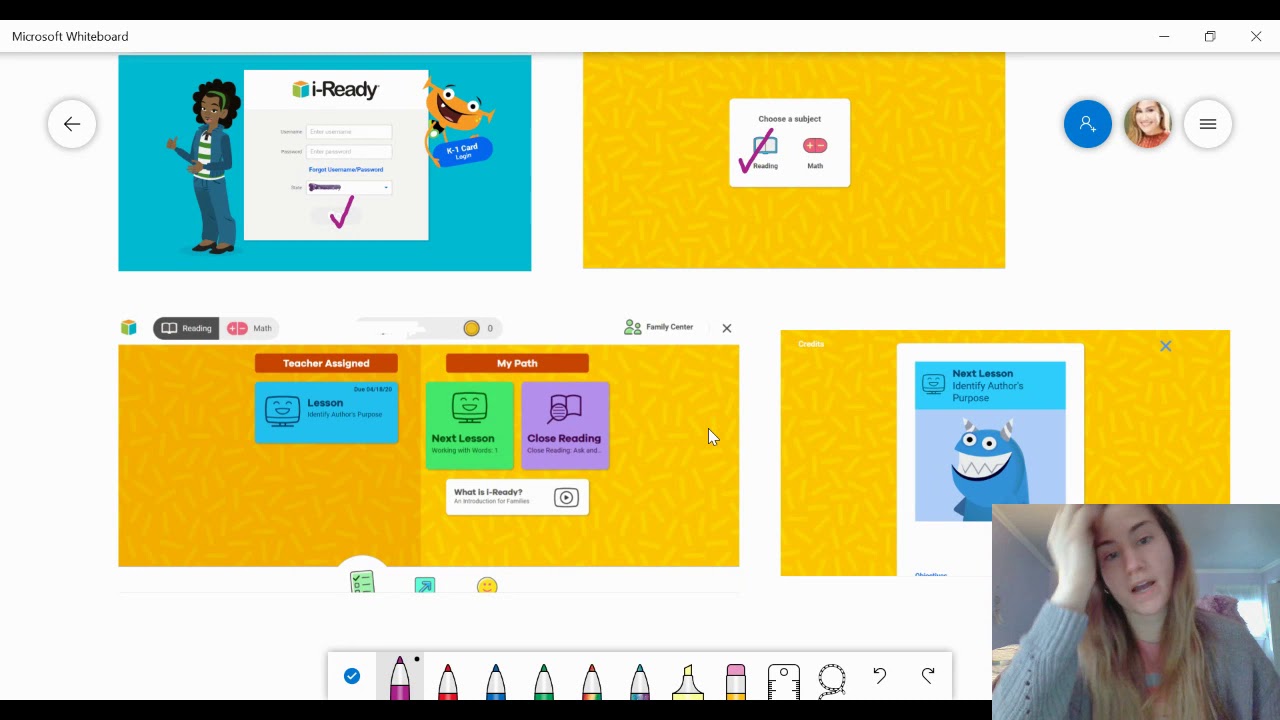This image is a screenshot of the Microsoft Whiteboard interface. The image features thin black lines at both the top and bottom, which frame the entire layout. 

Starting from the upper left corner, there is a white bar running horizontally across the top, with the phrase "Microsoft Whiteboard" written in black font. Beneath this bar, the main content is organized into separate sections. 

The first section, located in the upper left, is a box labeled "I Ready" displaying what appears to be a login screen. To the right of this box is a yellow box labeled "Choose a Subject." 

Directly below these two boxes are two additional boxes displayed side-by-side. The box on the left is labeled "Teacher Assigned," and beside it to the right, the box is labeled "My Path." 

Additionally, at the bottom right-hand corner of the screenshot, there is an inset image of a woman who appears to be a streaming person on a video call.